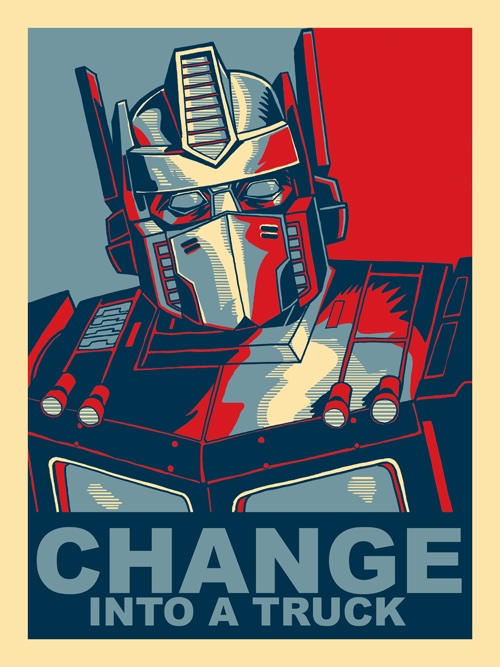This meticulously crafted color illustration is a parody of the iconic Shepard Fairey Obama poster, famous for its "Yes We Can" slogan. The artwork features a Transformer from the well-known toy and movie franchise, depicted as a colossal robot with a humanoid design. Utilizing a vibrant palette, the Transformer is adorned in striking shades of red, white, and blue. The background is split vertically, with the left half in blue and the right half in red, creating a stark contrast that emphasizes the central figure. Framing the image is a bold, dark yellow border. Positioned below the Transformer, rendered in blue text, is the humorous caption, "Change into a truck." This piece is purely illustrative, devoid of photographic elements, people, buildings, plants, animals, signs, or billboards, focusing entirely on its satirical homage to the original poster.